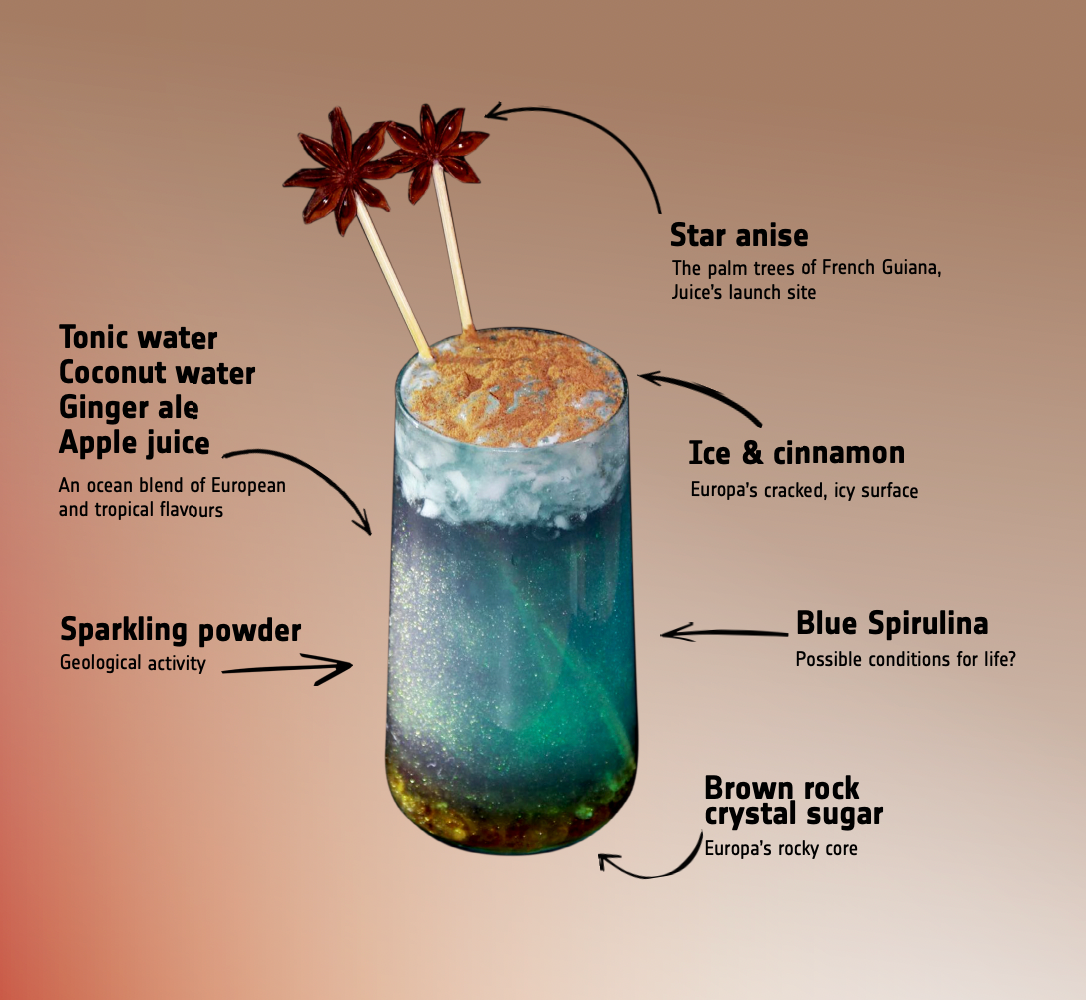The promotional-style poster features a detailed guide on crafting a vibrant and layered beverage, set against a light tan background. Central to the image is a cylindrical glass which tapers towards the top. This clear glass holds a striking drink layered from bottom to top in bluish-green, transitioning to white, and capped with a yellow, foamy layer. Floating in the drink, likely at the top, is ice sprinkled with cinnamon. Two long stirring sticks adorned with brown star-shaped star anise adorn the left-hand side of the glass.

Text around the image provides descriptive insights and ingredients. On the left, ingredients include tonic water, coconut water, ginger ale, and apple juice, labeled “an ocean blend of European and tropical flavors.” Below these, it mentions the addition of sparkling powder, suggesting “geological activity.” Arrows on the right label the brown stars on the sticks directly as "star anise, the palm trees of French Guiana Juice's launch site," hinting at an exotic flair. Another arrow points toward the top of the glass labeling the top layer as "ice and cinnamon," likened to "Europa's cracked icy surface." Just below, the vivid blue-green layer is identified as “blue spirulina, possible conditions for life?” Lastly, the very base of the drink contains “brown rock crystal sugar,” metaphorically referred to as “Europa's rocky core.” The artistic and scientific flair of the descriptive captions enhances the whimsical nature of this visually captivating beverage guide.